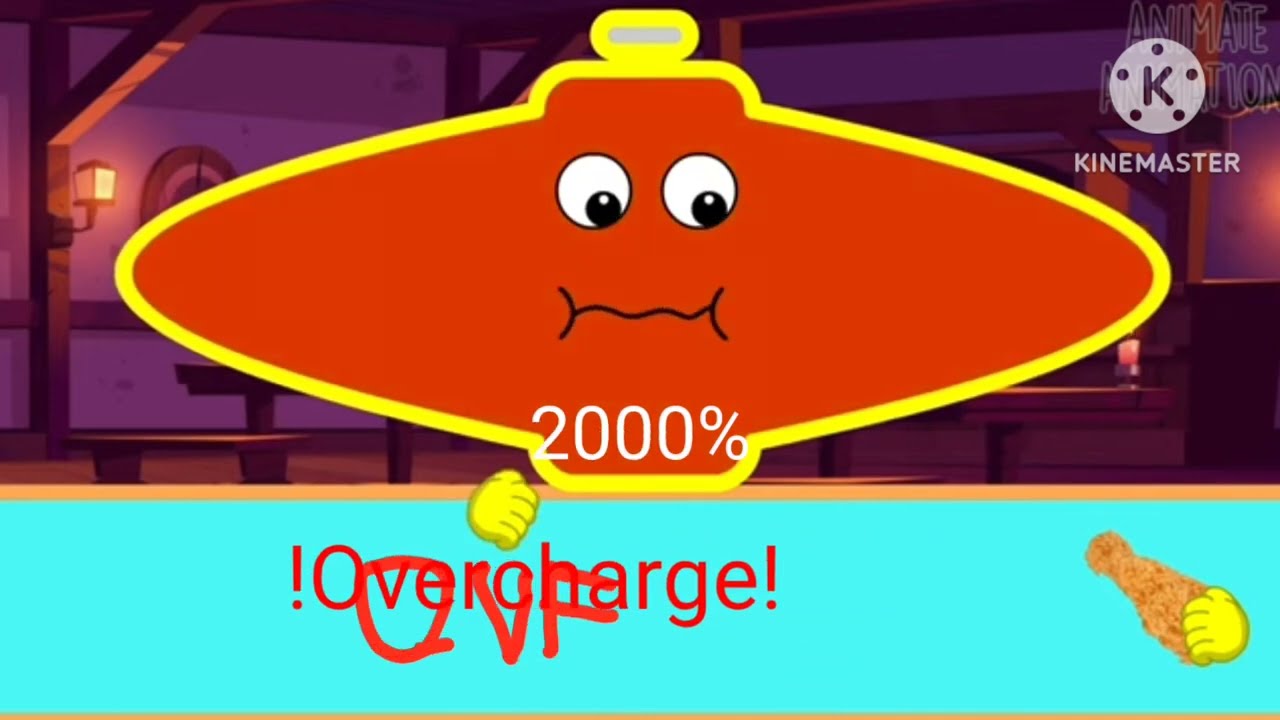The image depicts a brightly colored, cartoon-style scene that resembles a screenshot from a side-scrolling video game, set inside an animated castle or tavern-like interior. The background includes purple walls with brown vertical beams and lanterns emitting a warm, dim glow. On the left side, part of a dartboard is visible but partially obscured by the central figure. Dominating the center is a large, saucer-shaped cartoon character with a yellow outline and an orange interior. This character features two large eyes with black pupils and a wiggly mouth, giving it a sad expression. Below the character, in large white letters, is the text "2000%," and beneath this is a bright blue box with the word "OVERCHARGE!" in red letters flanked by exclamation marks. Additionally, the bottom right corner shows what appears to be a fried piece of food held by a yellow cartoon hand. The top right corner displays the text "Kind Master," likely referencing the program or application used to create the image.